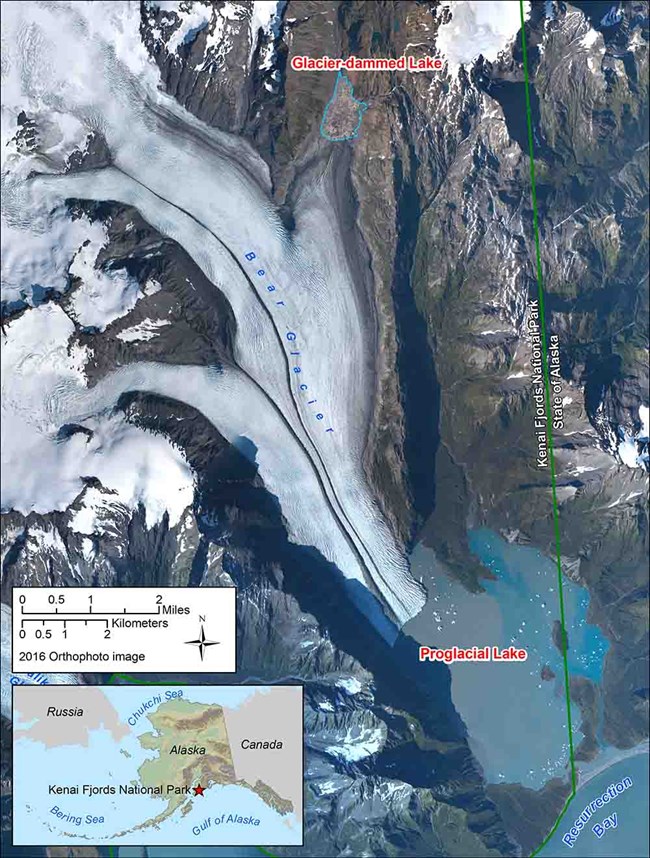This is an aerial orthophoto image from 2016 illustrating the Kenai Fjords National Park located on the southern coast of Alaska, near the Gulf of Alaska. The central focus of the image is Bear Glacier, which is depicted as a flowing white mass extending into the adjacent Proglacial Lake. Resurrection Bay is situated at the bottom right, while the Bering Sea can be seen at the very left of the image. A scale indicating miles and kilometers is present at the top of the picture, accompanied by a compass pointing north on the right side. A red star marks the location of Kenai Fjords National Park. The surrounding areas also feature labels such as Glacier Dammed Creek and various geographical markers. The context is secured by a thorough legend and labels indicating prominent landmarks, such as the Cheshire Sea at the top and the Gulf of Alaska at the bottom right.